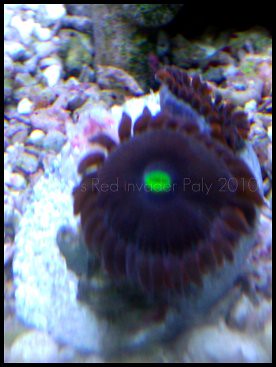The image depicts a reddish-brown and dark purple aquatic creature with a furry, tarantula-like texture. The creature, marked by a distinctive green dot on top, rests atop a prominent rock that is surrounded by other rocks of various colors, including light gray, blue, and pink. The surroundings suggest an underwater setting, further hinted by the presence of green fauna around the creature. There appear to be two of these creatures side by side. Imprinted over the image are the words "Red Invader Poly 2010," possibly identifying the species. In the upper left corner, the blurred image vaguely resembles tree branches.